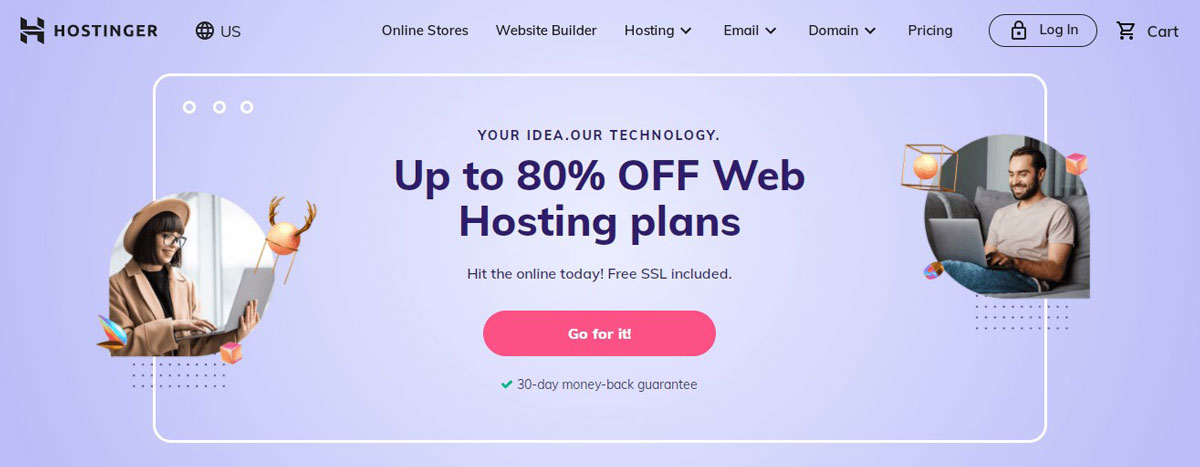This screenshot features the homepage of the Hostinger website. The background showcases a lilac gradient, which lightens towards the center, creating a visually appealing focal area. In the upper left corner, the Hostinger name is displayed in black font, accompanied by a stylized black "H" icon. Adjacent to it, a globe icon is paired with "US" in black font, indicating the selected region.

The navigation bar below includes several drop-down menus: Online Stores, Website Builder, Hosting, Email, Domain, and Pricing. To the right of these, there are buttons for Login and Cart, the latter marked by a shopping cart icon.

Centered beneath this navigation bar is a prominent white-outlined rectangle. Inside, the text "Your idea. Our technology. Up to 80% off web hosting plans. Hit the online today!" is displayed in black font. A pink button with white font below this message encourages users to "Go for it." Additionally, the text "30-day money-back guarantee" appears further down, accompanied by a small red checkmark. A promotional message, "Free SSL included," rounds off the offer, emphasizing added value for potential customers.